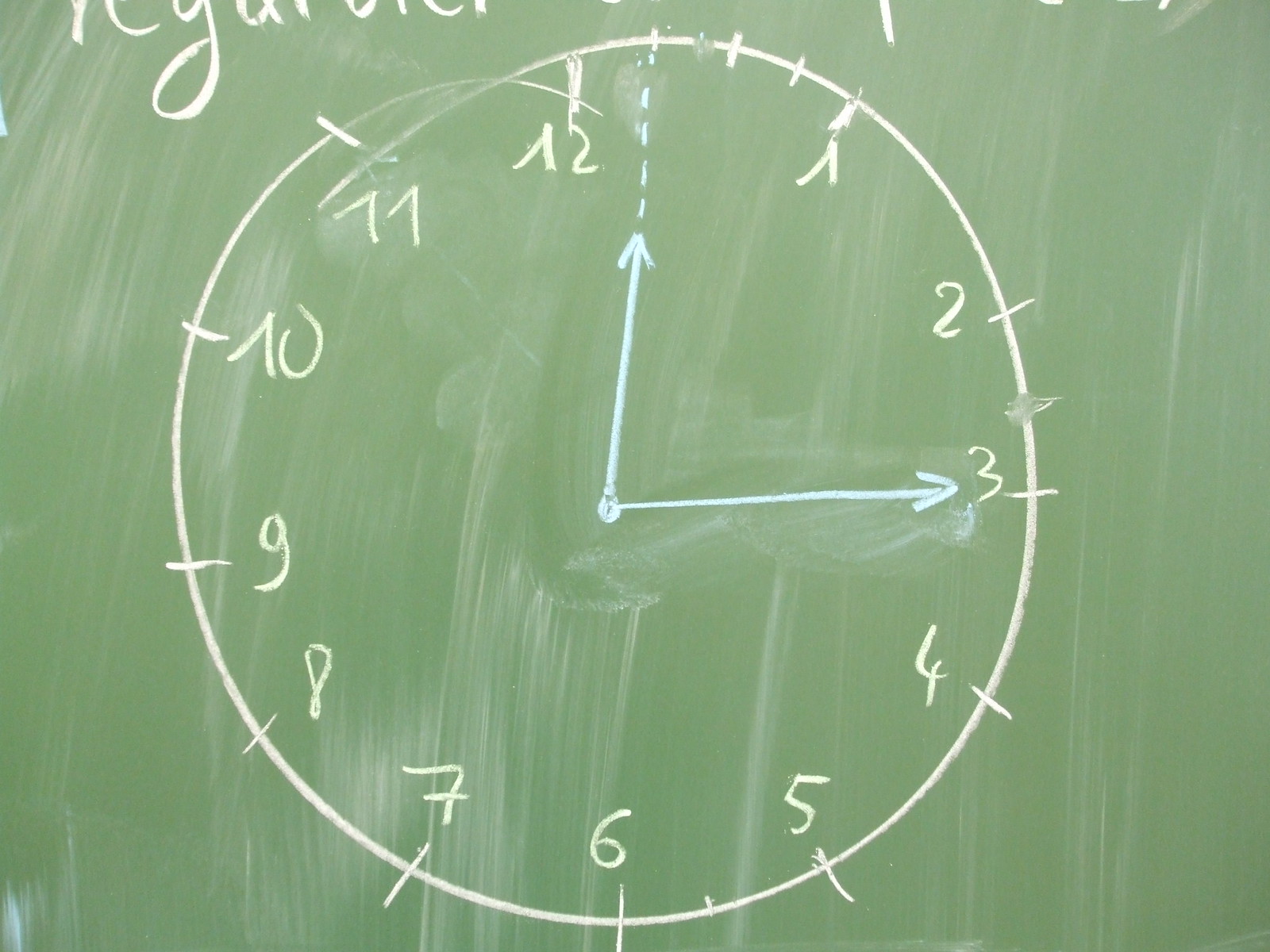The image depicts a chalkboard of sage green color, prominently featuring a hand-drawn clock face at its center. The clock, sketched in white chalk on a smeared background that shows signs of previous erasures, is not perfectly symmetrical. The numbers 1 through 12 encircle the clock face, but the number 12 has been corrected and is slightly askew. The clock's hour and minute hands are drawn in light blue chalk, with the hour hand pointing just past 12 and the minute hand at 3, indicating the time as 12:15. There are blue dashed lines extending from the hour hand upward towards the top of the clock face. Additionally, each hour is marked by white lines bisecting the circle, with smaller segments visible between the numbers 12 and 1. Above the clock, to the upper left edge of the board, there appears to be partially cropped, illegible writing in white chalk, contributing to the worn and reused appearance of the chalkboard.